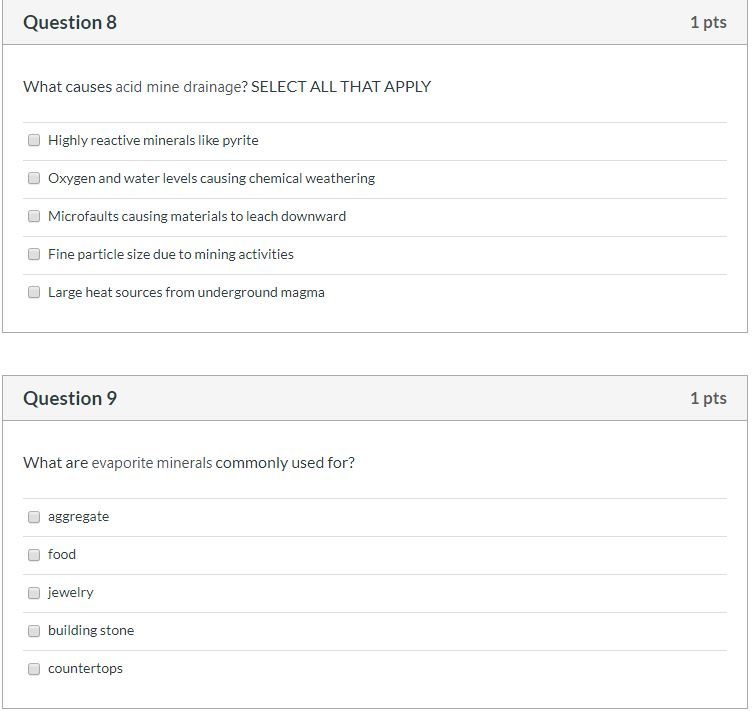The image shows a screenshot from an online quiz or survey, likely part of an educational platform used in high school or college classes. The screen displays two questions with multiple choice options. Question eight, worth one point, asks, "What causes acid mine drainage? Select all that apply." It provides five possible causes for participants to choose from. Question nine, also worth one point, asks, "What are evaporite minerals commonly used for?" Similarly, it lists five potential uses for respondents to select. Both questions suggest the context of an academic assessment focused on environmental science or geology topics.